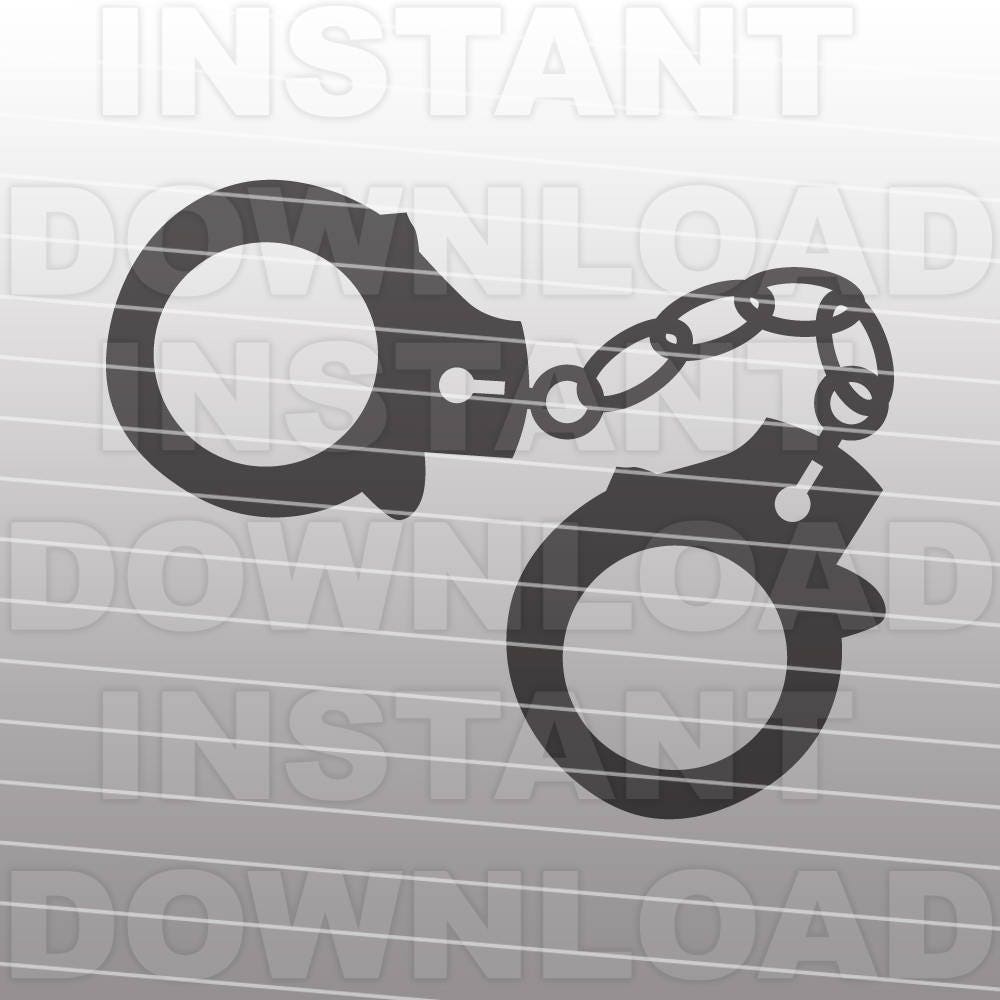This image is a flat, simple illustration of a pair of black handcuffs. Each cuff features a keyhole resembling a circle with a dash next to it and has a protruding locking mechanism. The handcuffs are linked by a circular ring, which connects to ovular rings that join the two cuffs together. The entire illustration is overlaid with diagonal white lines and a prominent watermark that repeatedly states "INSTANT DOWNLOAD" in large, capital letters. The watermark text is slightly slanted and spans across the image multiple times, indicating that this is a graphic available for immediate digital purchase and download.